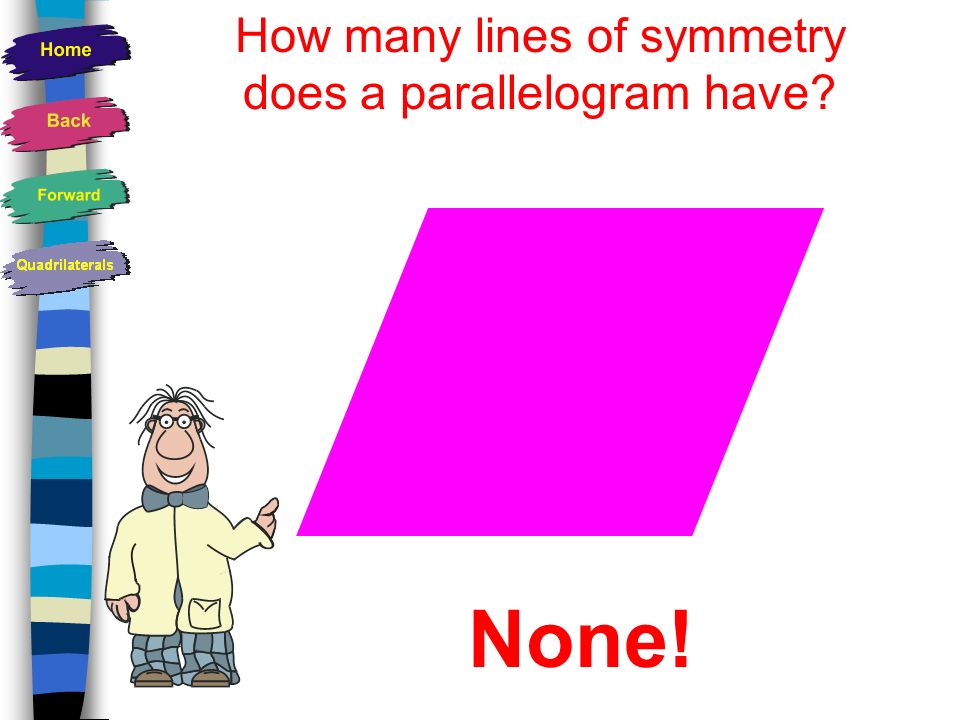The image appears to be an educational infographic, likely from an educational game or website. On the left side, there's a vertical stripe-menu in various shades of blue, black, off-white, and light yellow. At the top of the menu are four paint splash icons acting as buttons labeled "Home" (blue), "Back" (pink), "Forward" (green), and "Quadrilaterals" (light gray). To the right of this menu, a question in red text asks, "How many lines of symmetry does a parallelogram have?" Below the question is a pink parallelogram with the word "None!" written prominently underneath it. Adjacent to the parallelogram, on the left, is a minimalistic cartoon illustration of a professor or teacher, characterized by a white lab coat, gray bow tie, glasses, and curly hair, pointing at the geometrical shape. The overall design is clean and child-friendly, making it an effective tool for teaching geometry to young learners.